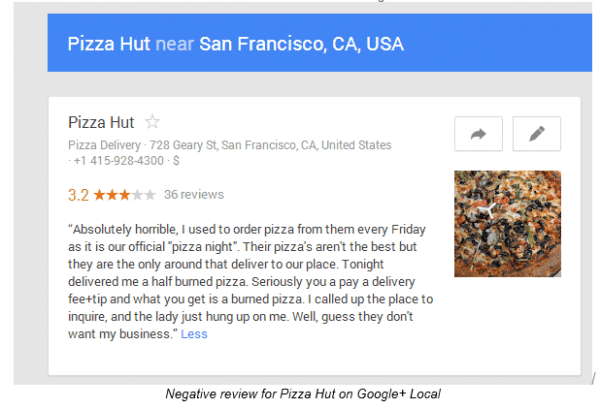**Negative Review for Pizza Hut on Google Plus Local**

**Location:** Pizza Hut, near San Francisco, California, USA

**Description:**
A review for Pizza Hut located at 728 Kearny Street, San Francisco, California, United States. The listing is marked with white text in a blue box, highlighting "Pizza Hut" near the top. The establishment is categorized under "Pizza Delivery" and has a contact phone number of 1-415-928-4300, displayed alongside a single dollar sign indicating pricing. 

**Ratings and Reviews:**
- **Overall Rating:** 3.2 out of 5 stars based on 36 total reviews.
- **Recent Review:** 
  - **Rating:** 1 star
  - **Comment:** "Absolutely horrible. I used to order pizza from them every Friday, as it is our official pizza night. Their pizzas aren't the best, but they are the only ones around that deliver to our place. Tonight, they delivered me a half-burned pizza. Seriously, you pay a delivery fee plus a tip, and what you get is a burned pizza. I called up the place to inquire, and the lady just hung up on me. Well, guess they don't want my business."

**Visual Elements:**
- To the right of the review details, there are two icons: an arrow pointing to the right and a pencil.
- A photograph is included, presumably showing the burned pizza received by the reviewer.

This detailed caption presents the essential aspects of the negative review, providing context and highlighting the negative customer experience.